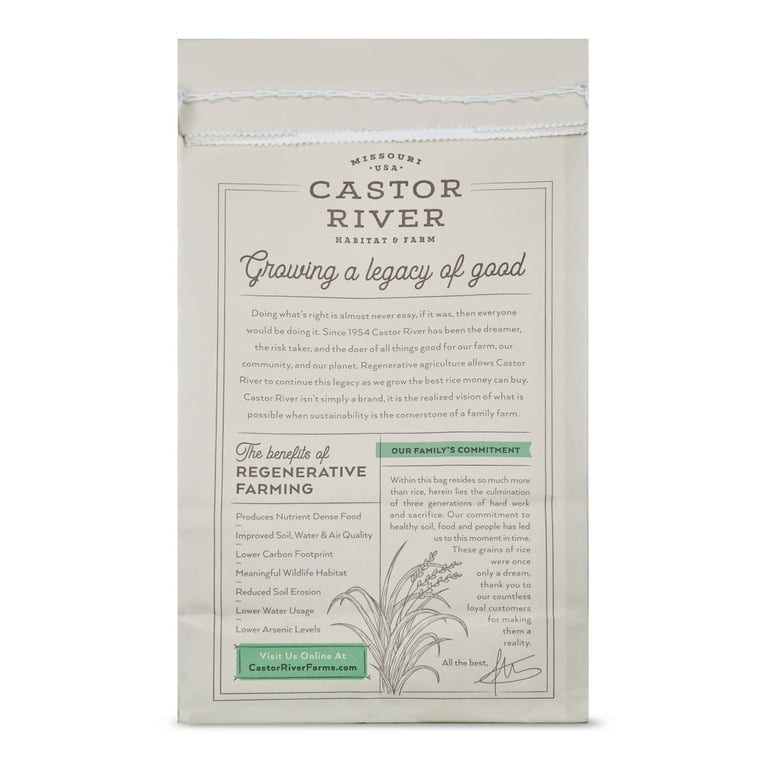The image depicts the back of a soft, brown paper packet that provides detailed information about regenerative farming and Castor River Habitat and Farm in Missouri, USA. At the top, bold black font reads: "Castor River Habitat and Farm, Missouri, USA. Growing a legacy of good." Directly beneath this header is a small paragraph of text. The packet's layout features several sections and columns, including "The Benefits of Regenerative Farming" and "Our Family's Commitment," each accompanied by text and bullet points. At the bottom left, there's a green box with the text: "Visit us online at castorriverfarms.com." An illustration of a plant with long, curved leaves is at the center bottom, and a handwritten signature appears in the bottom right.